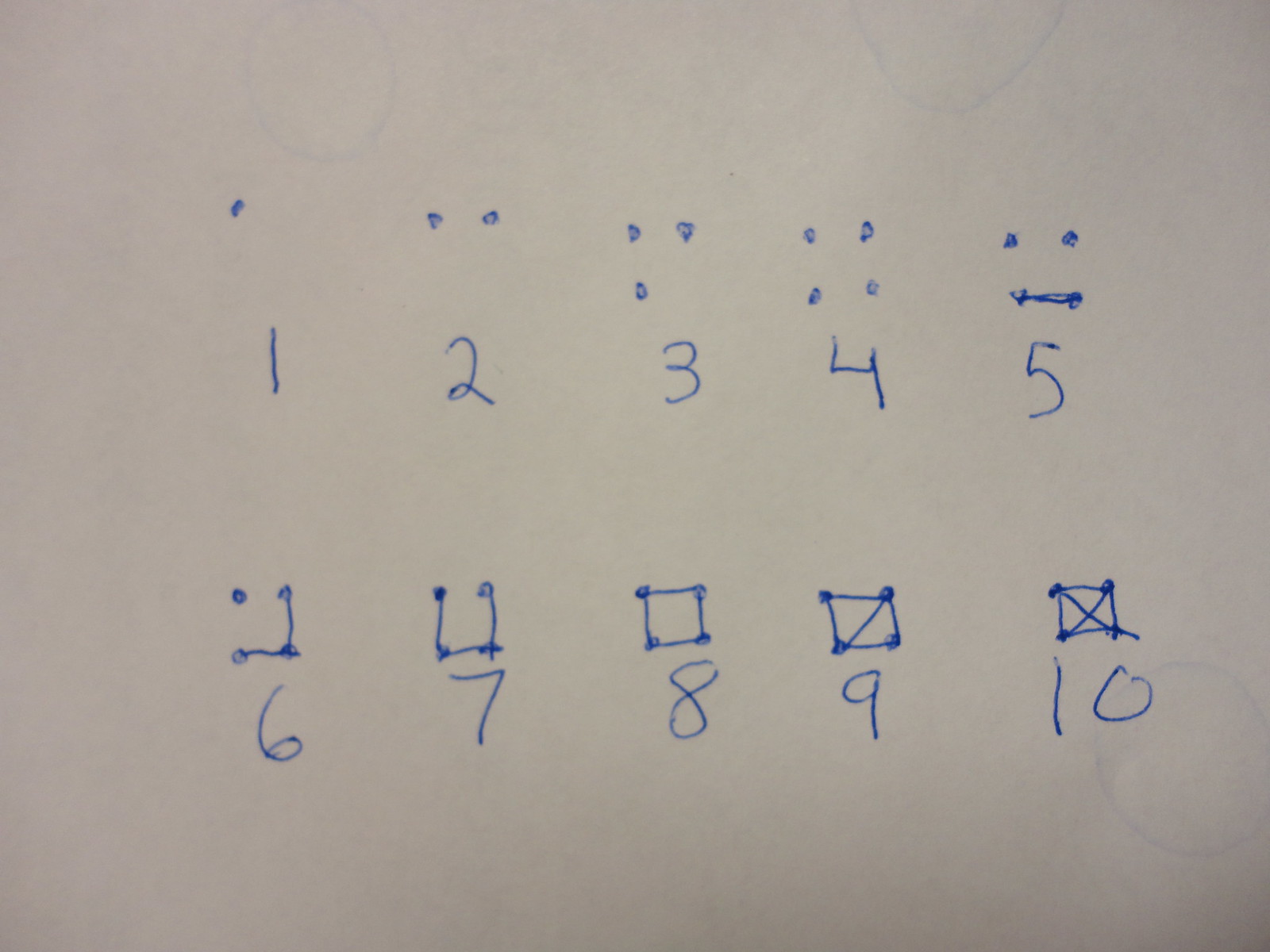In the image, there is a drawing on brown scrap paper, which appears to be part of a lesson or educational game focused on numbers and dots. The illustration showcases the numbers 1 through 10, each adorned with a unique arrangement of dots and lines above them. 

- Number 1 has a single dot above it.
- Number 2 has two dots aligned horizontally.
- Number 3 has three dots aligned vertically.
- Number 4 features four dots arranged in a square pattern.
- Number 5 uses the same four dots in a square with an additional horizontal line below them.
- Number 6 builds upon the previous arrangement by adding a vertical and horizontal line to the right side of the bottom two dots.
- Number 7 adds to this configuration by incorporating an additional vertical line on the left side, forming a 'U' shape around the four dots.
- Number 8 encloses the four dots entirely with lines, creating a complete square.
- Number 9, similar to the previous square, includes a diagonal line from the bottom left to the top right across the square.
- Number 10 features the complete square with both a diagonal from bottom left to top right and an additional diagonal from top left to bottom right, forming an 'X' inside the square.

The detailed configurations help illustrate the numerical values and their corresponding dot patterns vividly.